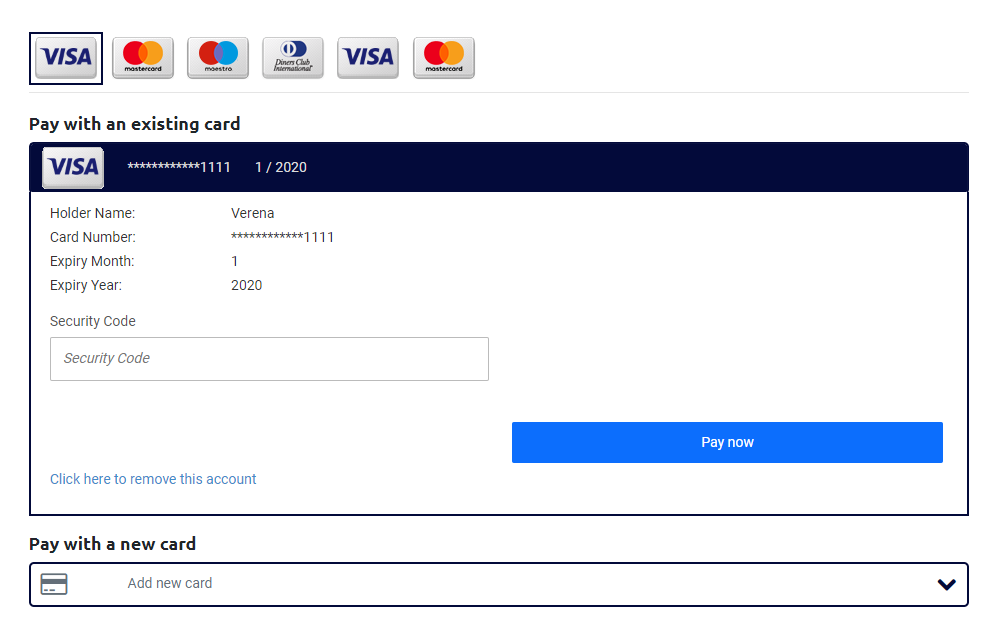In this detailed screenshot of the payment screen on an unidentified website, users are presented with the option to complete a transaction using various card types. The upper section of the interface displays recognizable symbols for different credit card brands, notably Visa and MasterCard. The cardholder, named Verena, is in the process of using her Visa card, with details like the card number ending in "1111" and an expiration date set for January 2020 already inputted.

The form includes fields for additional information, such as the security code, which Verena has not yet filled out. Since this is an existing card saved on the account, there is a visible option labeled "Click here to remove this account." Furthermore, a prominent blue "Pay Now" button is available for finalizing the payment once all necessary information is entered. Additionally, the interface offers the option to "Pay with a new card," allowing users to input details for a different card if desired. Verena, however, has chosen to proceed with her pre-saved Visa card instead of entering a new one.